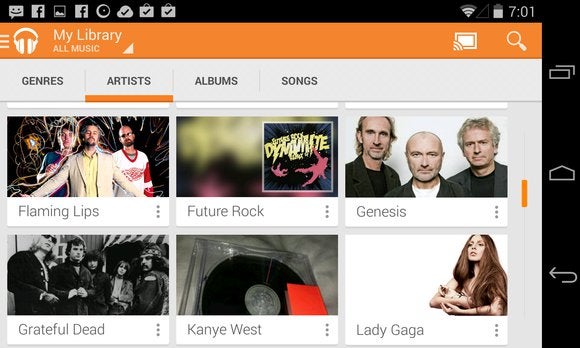This image is a detailed screenshot taken from a website or mobile device, showcasing the user's music library. At the top of the screen, an orange banner prominently displays the title "My Library." Just below this title, the words "All Music" appear alongside a headphone icon on the left side of the banner.

Directly beneath the banner, four categories are listed in a horizontal row: Genres, Artists, Albums, and Songs. The "Artists" category is highlighted, as indicated by an orange bar underneath it.

The main body of the page features a grid layout of artists, consisting of six different artist icons arranged in two rows and three columns. Each icon includes an image of the artist or band members, with the artist's name displayed below the image. 

On the first row, from left to right, the artists are:
1. The Flaming Lips
2. Future Rock
3. Genesis

On the second row, from left to right, the artists are:
1. Grateful Dead
2. Kanye West
3. Lady Gaga 

Each image is in color, giving a vibrant and visually appealing look to the library's interface.